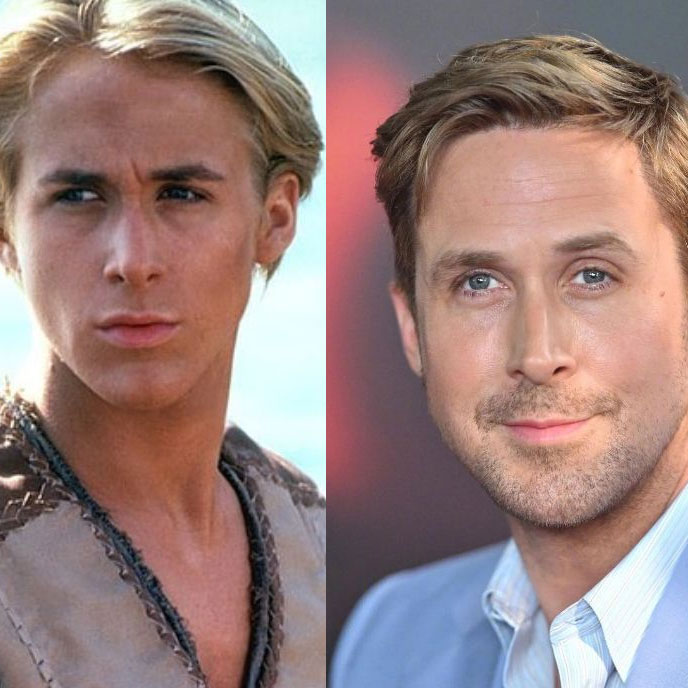The image consists of two side-by-side photographs of Ryan Gosling at different stages in his life. On the left is a younger Gosling, possibly in his early 20s and starring in a film. He has a clean-shaven, gaunt baby face, with blonde hair and normal-sized ears. He is wearing a dystopian sci-fi outfit, reminiscent of "Dune," that is brown with darker brown trim and exposes part of his chest. The background appears to be a solid blue.

On the right is a more recent paparazzi photo of Gosling, taken at a premiere when he is in his mid-30s to early 40s. In this image, his hair is a darker blondish-brown, and he sports light stubble over his lips and chin. His blue eyes are highlighted against his blue dress shirt and jacket, and his lips are a noticeable pink. The background features a blurred mix of gray and pink tones. Both photographs are cropped to show Gosling from the chest up.